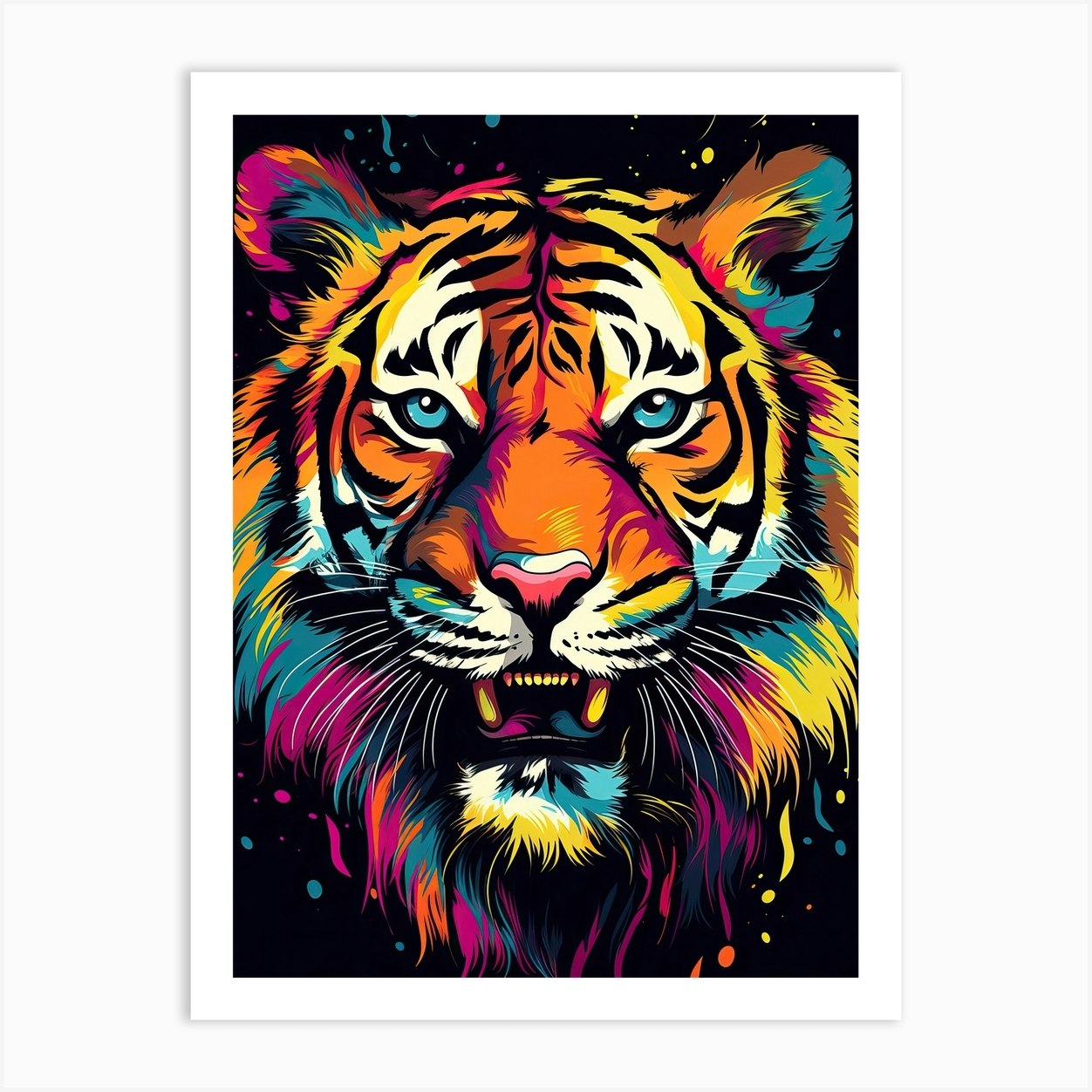This is a highly detailed and vibrant graphic art print poster of a tiger that fills about 95% of the composition, leaving just a hint of a black background adorned with colorful paint splatters. The tiger's head is the sole focus, depicted with meticulous attention to detail and artistic liberties. While retaining the classic orange, white, and black stripes, the tiger’s fur bursts with a spectrum of vivid colors including purples, blues, yellows, pinks, and even hints of brown. The eyes are a piercing blue, and it gazes directly at the viewer, with its mouth open in a fierce snarl, revealing sharp, yellow fangs and hot pink and blue lips and tongue. The black background is delicately splotched with the same vibrant hues found in the tiger's fur, enhancing the overall dynamic and striking appearance of the artwork. The diverse and lively color palette makes this piece a captivating addition to any room, particularly appealing as an inspiring decoration for a teenager's space, encouraging creativity and artistic expression.